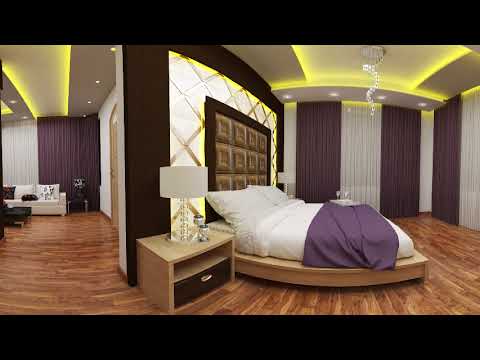This image captures a luxurious bedroom suite, likely in a high-end hotel. The centerpiece of the room is a bed adorned with a white comforter and a purple blanket, set against a dark brown, waffle-pattern headboard with a matching brown frame. The bed has light brown wooden supports and is accompanied by white sheets and pillowcases. On either side of the bed, there are wooden nightstands, each topped with clear glass lamps with white shades. The floor is covered in rich, dark hardwood that extends into an adjacent living room area.

The room is well-lit with a mix of bright yellow ceiling lights and recessed can lights, complemented by a distinctive spiral chandelier. Both the bedroom and the adjoining living area feature purple and white curtains and a white couch. The ceiling is white with yellow trim, creating a warm ambiance that enhances the suite's elegant design. Overall, the room exudes a sophisticated and cozy atmosphere.